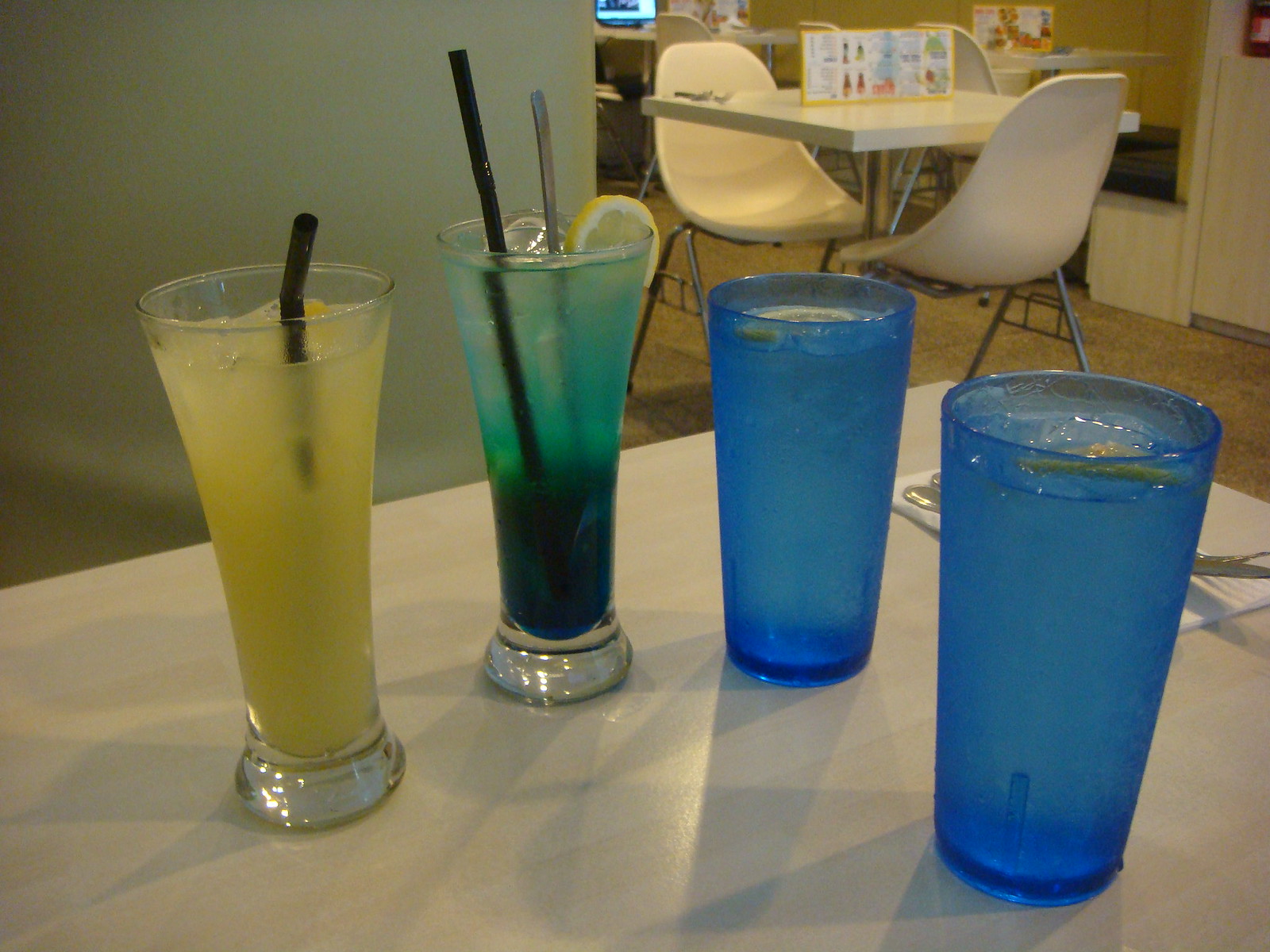The vibrant color photograph captures a cheerful and colorful scene focused on a white table in the foreground. At the center of attention are four distinctly different drinking glasses. Positioned on the left side are two tall Pilsner-like glasses: the leftmost glass contains a yellow lemonade-like beverage with ice and a black straw, while the adjacent glass holds a bluish-green liquid, garnished with a lemon wedge and featuring two black straws. On the right, two medium translucent blue plastic tumblers are visible, each filled with water, ice, and a floating lemon slice. Also on the table is a paper napkin with a knife and fork neatly placed beside the blue tumblers.

In the background, the image reveals a square white table adorned with a standalone menu, flanked by two molded fiberglass chairs reminiscent of Eames-style seating. The background setting includes a white wall on the left and a hint of a TV or monitor in the upper section. The floor appears to be brown tile, reinforcing the casual, homey ambiance of the room. The overall composition of the photograph presents a vivid and inviting snapshot of a cheerful dining or kitchen area.